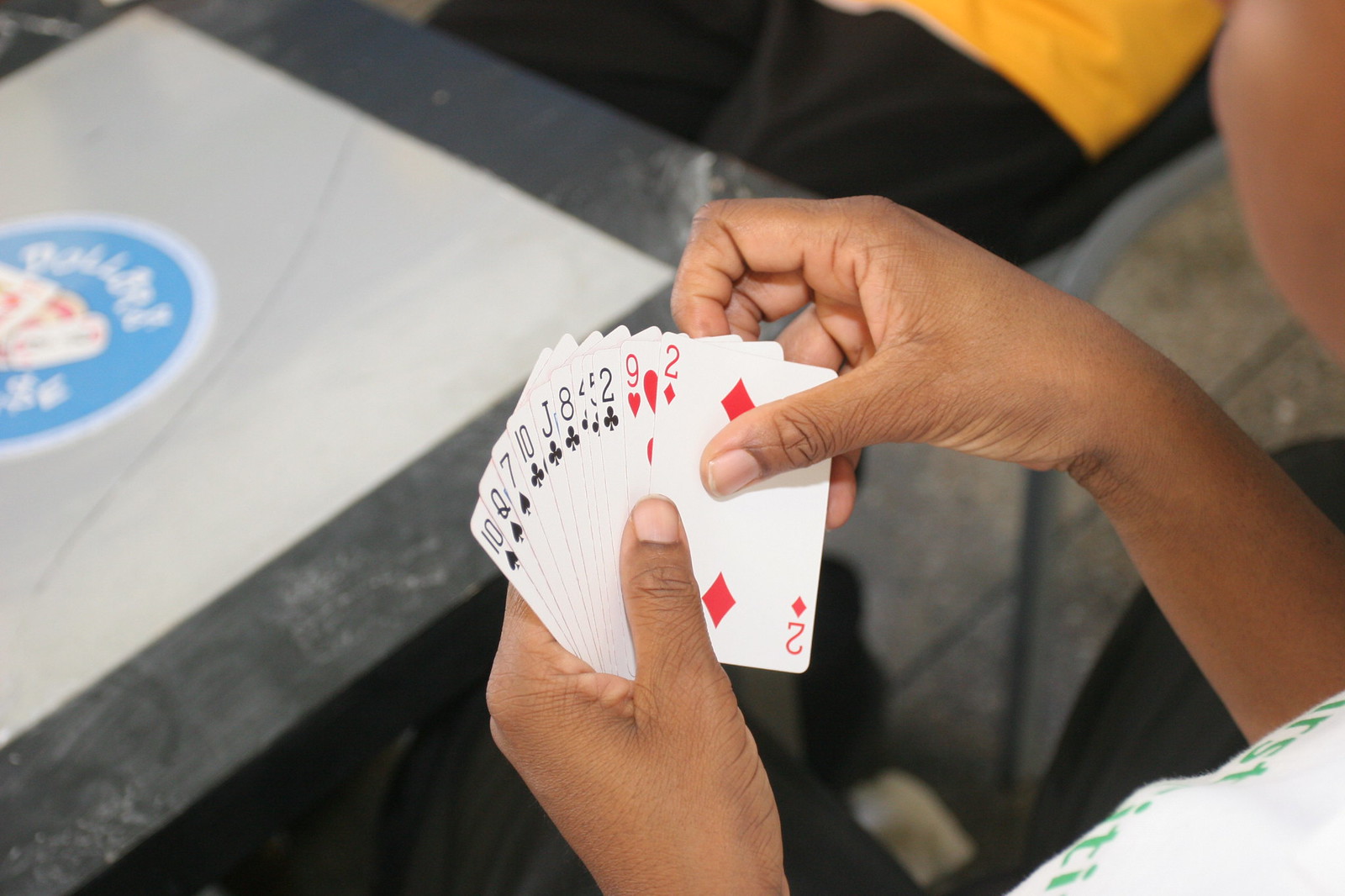A person is captured holding a fan of playing cards in one hand. In the bottom right corner, part of their white shirt with indiscernible green lettering is visible. Their other hand is positioned above the cards, showing the inside of the forearm and thumb, and partially concealing the fingers as they grip the cards. A small portion of their face, notably the cheek, is visible in the upper right. Beyond the face, the ground beneath them is gray. To the left, a yellow shirt, black shorts, and a gray chair with a black seat come into view slightly.

The cards are spread out in a neat fan, displaying from left to right: the 10 of spades, queen of spades, 7 of spades, 10 of clubs, jack of clubs, 8 of clubs, 4 of clubs, 5 of clubs, 2 of clubs, 9 of hearts, and 2 of diamonds. The background includes a gray table, light gray in the center with a darker gray border, extending from the left corner to the bottom right. A blue circle with a light blue trim and indistinguishable white lettering appears near the center, partially extending off the side of the image.